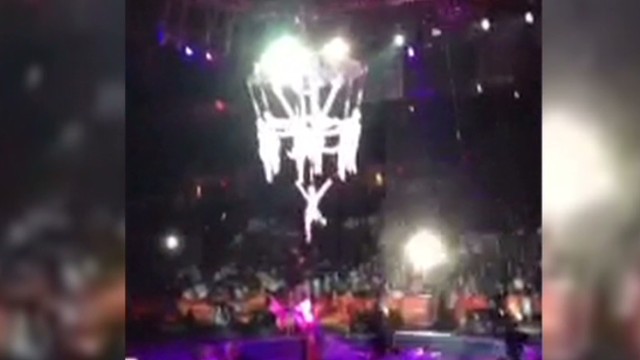The image portrays a concert stage bathed in vibrant purple and pink lights, set within a large stadium. Above the stage hangs an elaborate, bright white fixture that captivates the eye with its glowing intensity but is too luminous to reveal its intricate details clearly. Suspended around the periphery of this fixture are several people arranged in a circular formation. Central to this aerial display, one individual hangs the lowest, striking a dynamic pose with one leg extended forward and both arms reaching skyward. The audience gathers densely around the stage, adding to the electric atmosphere, while additional lights beam down from above, illuminating the entire scene in a captivating blend of colors.